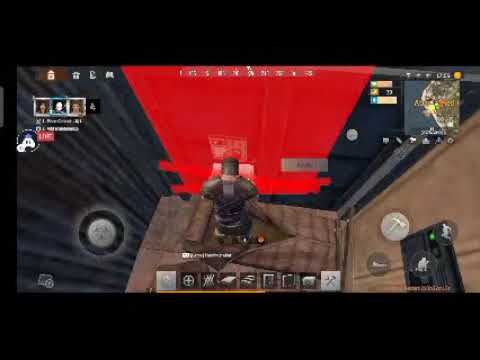In this detailed screenshot from an action-adventure video game, the central scene showcases a soldier clad in a brownish-green helmet and matching shoulder pads, bent over and seemingly examining an object on the ground, perhaps a book. The surroundings suggest the interior of a moving van, characterized by metal sheet walls. Directly in front of the character is a dominant red wall, and adjacent to it is a beigeish-brown sleeping bag paired with a brown pillow laid out on the floor.

The interface is rich with details. At the top of the screen, a compass bar indicates cardinal directions. On the top right, a small, distinct mini-map shows the player's location, possibly with team member health or status displayed around it, indicating a multiplayer aspect. The bottom part of the screen features control icons—one symbolizing a jumping character, another a crouching figure, and additional icons like a hammer and a horn. The bottom center presents a series of nine selectable options, perhaps part of a start or inventory menu.

To the left, an interface shows a joystick symbol for character movement, while in the top left corner, there are three character icons next to a microphone, suggesting voice chat functionality. An array of weapon icons below the main character includes a shield, an axe, books, and stone. On the right wall, a circle with a hatchet symbol is visible, while the left wall bears a planetary icon within a circle. This complex overlay and the setting suggest a scenario where the player is deeply immersed in navigating, strategizing, or equipping the character within the game.